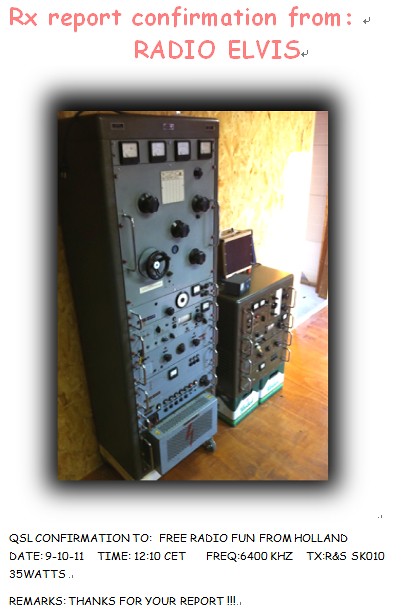The image displays vintage radio machinery set against a wooden plywood wall with a wooden floor. Dominating the scene is a tall, dark gray metal radio unit, notably about twice the height of the adjacent smaller light gray unit to its right. Both units are equipped with numerous handles, buttons, knobs, and switches, indicating complex functionality. The taller unit appears mobile, possibly mounted on wheels, while the smaller unit features a noticeable screen on top. The image itself has a black glow and is presented on a white background with vibrant red-pink text above it stating: "RX reports confirmation from Radio Elvis." Below the machinery, the caption reads: "QSL confirmation to Free Radio Fund from Holland, date 9-10-11, time 12:10 CET, frequency 6400 kHz, TX, RN, RNS, SK010, 35 watts, remarks: thanks for your report."